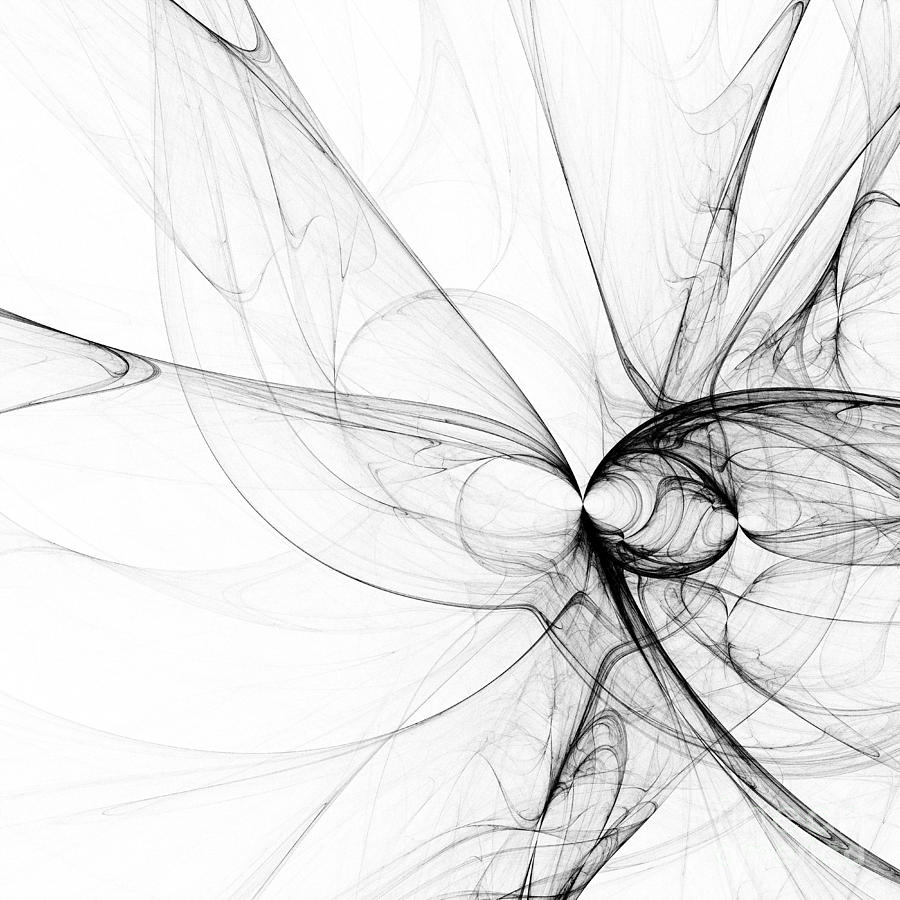This computer-generated artwork features a striking abstract design predominantly in black set against a contrasting white or light gray background. The central focus of the piece is a dense, dark black area located towards the right side of the image. From this focal point, intricate, veil-like lines and swirls emanate outward, creating a complex pattern reminiscent of ink dropped in water or designs produced by Spyrographs. These lines spread across the image in various directions, imparting a sense of fluidity and motion. The darker areas near the center suggest the delicate structure of insect wings, possibly resembling a butterfly, although the form is obscured by overlapping lines and swirls. As the lines extend further from the center, they lighten to various shades of gray, giving the impression of a gradual dispersion of ink. The overall composition is both detailed and delicate, evoking a sense of ethereal beauty and abstract form.